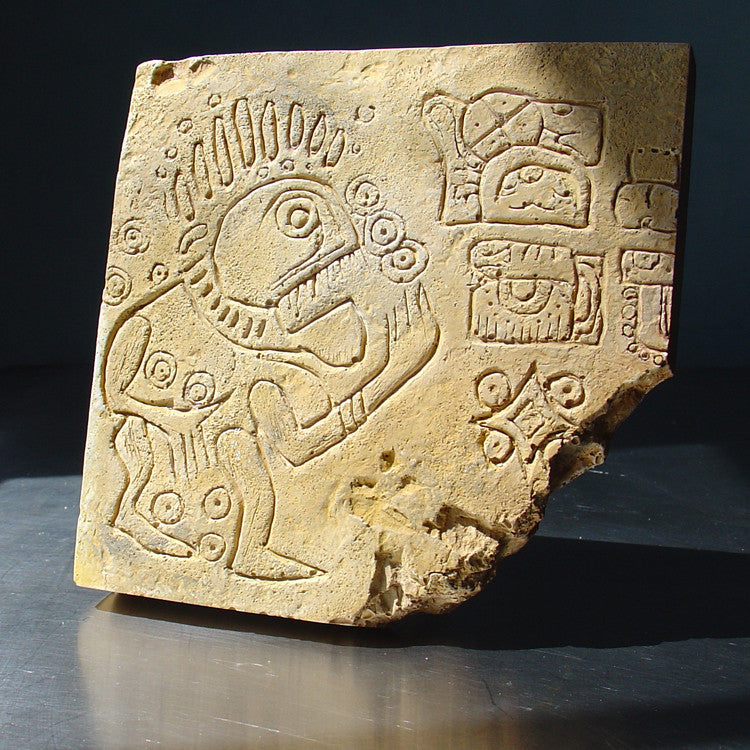This image features an angled view of a sandstone-colored, porous stone tablet with intricate carvings. Dominating the center-left of the tablet is a menacing creature with tall, spiky hair, one visible eye, and a mouth full of sharp teeth. The creature is depicted in a side profile, juggling round objects in its left hand while more of these objects are held and dropped by its right hand. The creature appears to be wearing a choker and a crown, adding to its threatening appearance. To the right of the creature, the tablet features various geometric designs, including circles, semicircles, triangles, and rectangles. Additionally, there are carvings of a star shape with rounded edges, a couch, a briefcase or suitcase, and a diamond shape. The tablet is intact except for the bottom right corner, which is broken off, and the upper right corner casts a shadow. The stone is placed on a shiny gray surface, enhancing the intricate details of the carvings.